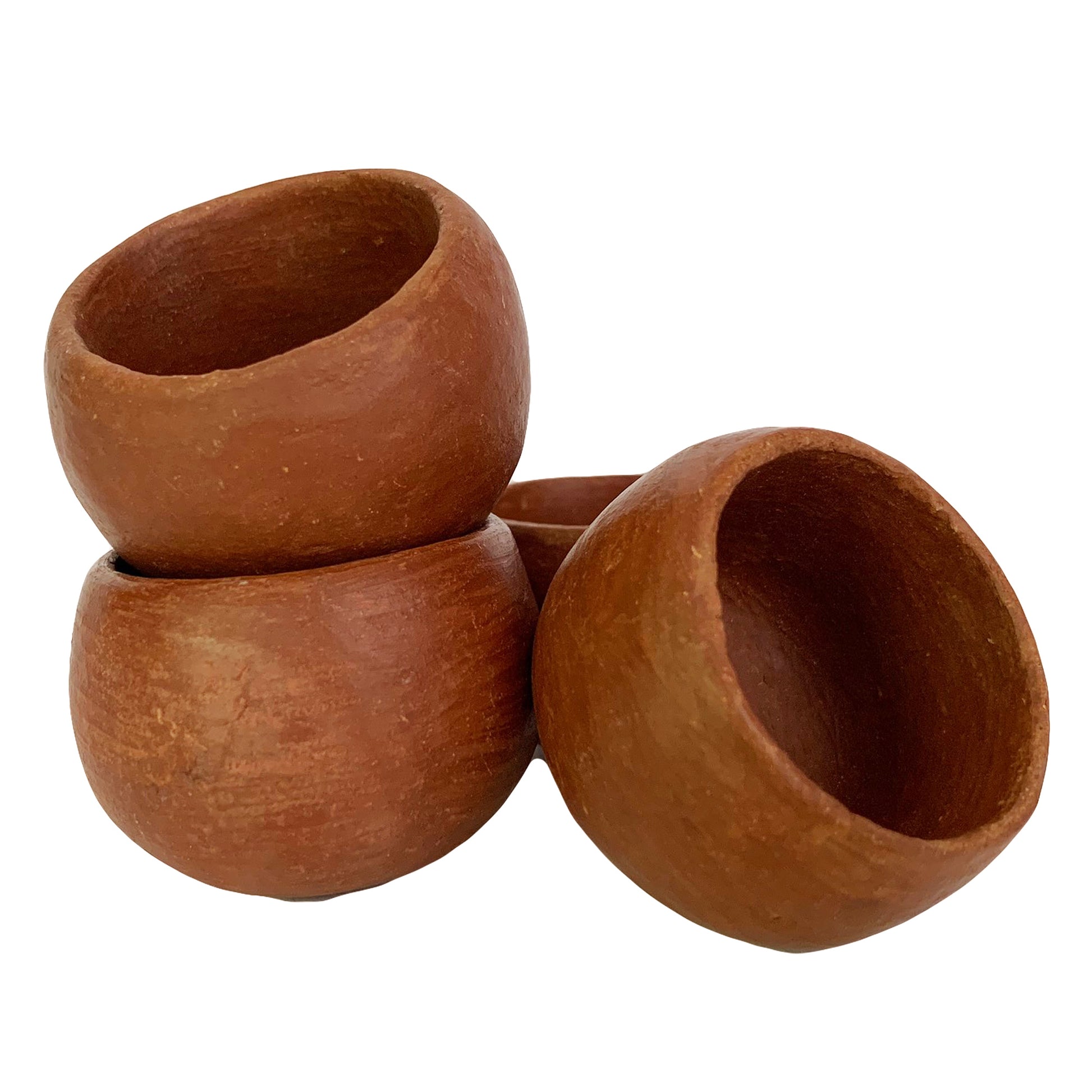This is a close-up, full-color photograph of four small handmade bowls arranged against a white background. The bowls vary slightly in shape, size, and shade, suggesting they are crafted from terracotta, giving them an orangey-red color, although some descriptions hint at a darker, wood-like brown. The textured bowls exhibit imperfections that add to their artisanal charm. In the arrangement, two bowls are placed flat on their base, with one bowl slightly tilted and leaning against the other two at the front. On the left, one bowl is stacked on top of another, both slightly tilted towards the left. The fourth bowl is positioned at the back, with only its lip visible. The simple, clear setup showcases the rustic beauty of the bowls, likely intended to illustrate an item for sale.